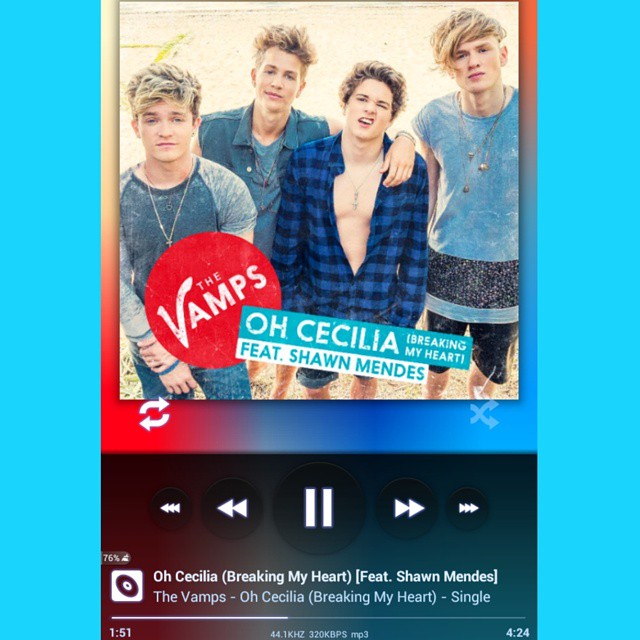The image is a detailed screenshot from a music streaming app. At its center, there's an album cover featuring four young men with a mix of blonde and brown hair, posing together on a beach. They're casually dressed in shades of blue, both short and long-sleeved shirts, with a youthful and relaxed appearance. Behind them, the sand and sky emphasize the summery vibe. Prominently displayed over the photo is a bold red circle with white vertical text that reads "The Vamps," indicating the band's name. Below the photo, an off-kilter blue sign highlights the song title, "Oh Cecilia, Breakin' My Heart," featuring Shawn Mendes, with some parts of the text in capital letters for emphasis.

Below this, there are traditional music player controls, including forward, backward, and pause buttons, alongside a progress bar. The text under the controls repeats the song title and the featuring artist, affirming it as a single titled "Oh Cecilia, Breakin' My Heart." Time indicators show that the song is 4 minutes and 24 seconds long, with the current playback position at 1:51. The overall background of the app screen is aqua blue, which frames the album cover and control section, making the band members' images stand out. The app interface suggests it is user-friendly with clear visual markers for song navigation and playback.